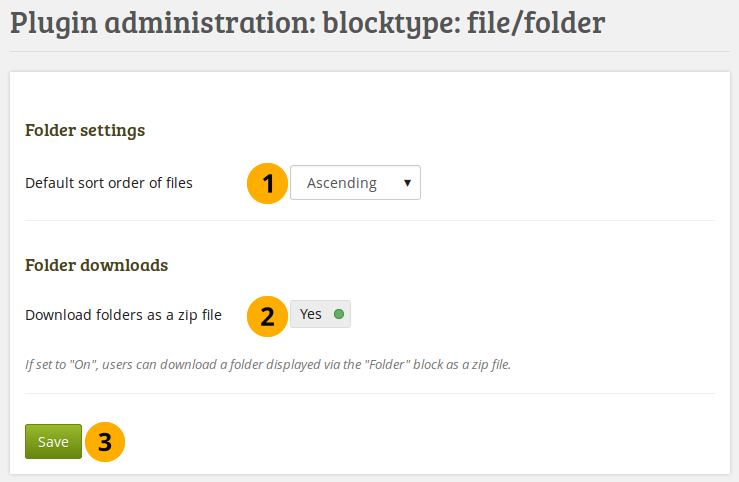The image displays a web interface for plugin administration, specifically focusing on the 'Folder Settings' options within a certain file or folder management system.

The overall layout is organized within a predominantly gray border:

1. **Top Section:**
   - The top contains a menu approximately two inches thick that reads in black text: "Plugin Administration, Block Type, File/Folder."
   
2. **Middle Section:**
   - Beneath the header is a thin gray line separating the top menu from the main interface.
   - The main interface is a white box:
     - **Upper Left Corner:**
       - Black text titled "Folder Settings."
       - Below this, it says "Default Sort Order of Files."
       - To the right of this text is a yellow circle containing a black number '1'.
       - Adjacent to the circle is a dropdown bar in white with black text that reads "Ascending" followed by a downward arrow.
       - A thin gray line separates this section.

     - **Folder Download Settings:**
       - The text "Folder Download" in black is below the gray line.
       - Underneath, it reads "Download folders as a zip file."
       - Next to this text, to the right, is another yellow circle with a black number '2'.
       - To the right of the circle is a gray switch labeled "Yes" in black text.
     
3. **Bottom Section:**
   - This section contains the instruction, "If set to 'on', users can download a folder displayed via the 'Folder' block as a zip file."
   - Below this, a green bar with the word "Save" in white lettering is located at the bottom.
   - To the right of the green bar is another yellow circle featuring a black number '3'.

The components are structured clearly to guide users through setting folder options, complete with numbered indicators for each step of the process.